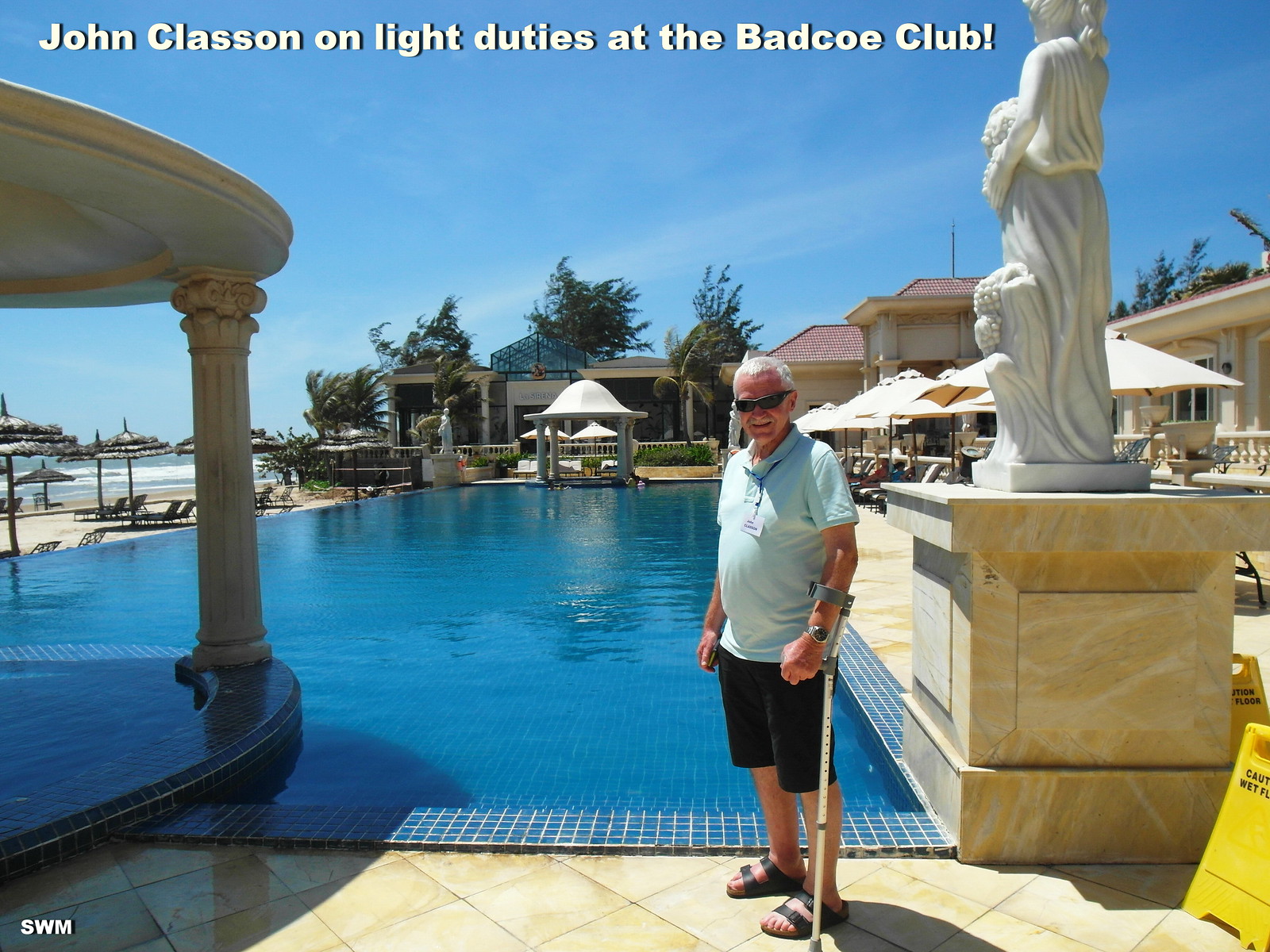This photograph captures an elderly man standing in front of a vibrant, blue pool on a beautiful, sunny day. He is wearing a light blue polo shirt, black shorts, sandals, and black sunglasses. The man, who has white hair, uses a cane attached to his left arm with a brace, hinting at a possible injury or disability. Despite this, he is smiling cheerfully. Behind him, the expansive pool dominates the middle of the image, extending towards a background dotted with patio coverings and a stone pedestal adorned with a statue of a woman facing away. The sky above is a clear blue, and strong winds are evident as the branches of trees in the background are noticeably blown to the right. To the left, one can also spot the tops of some trees and buildings. In the far distance, beach chairs arrayed on a short sandy beach suggest that the ocean isn't far from this tranquil pool area. Additionally, the caption at the top identifies him as John Klasson, noting he is on light duties at the Bad Co. Club.